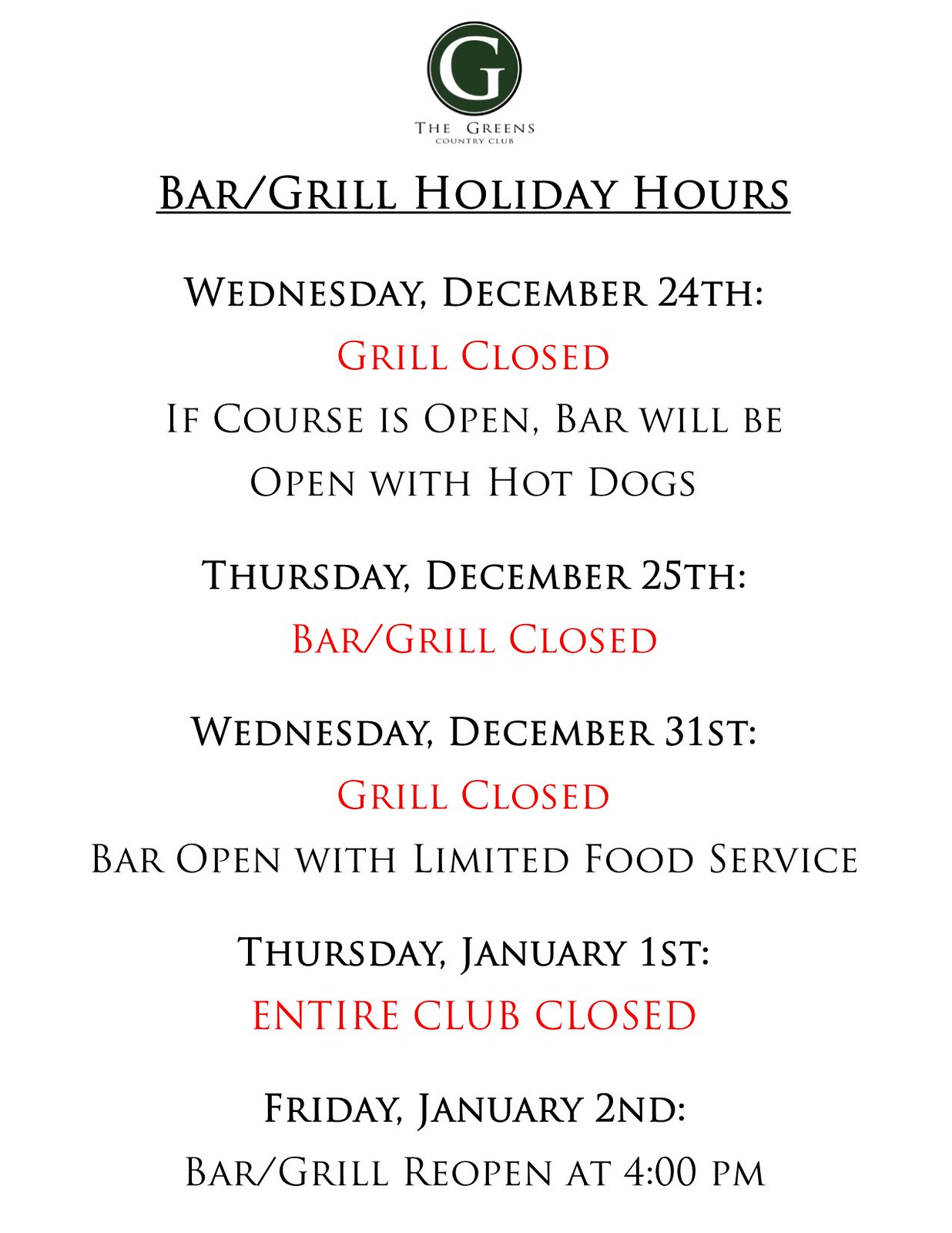The image is an informational flyer detailing the holiday hours for the Bar and Grill at The Greens Country Club, set against a completely white background. At the very top, a green circle featuring a large, white capital letter "G" is prominently displayed. Directly below this is the name of the establishment, "The Greens Country Club," in black text. The main body of the flyer features bold text stating "Bar/Grill Holiday Hours." 

Following this heading, the specific holiday hours are listed:

- **Wednesday, December 24th:** Grill closed. If the course is open, the bar will serve hot dogs.
- **Thursday, December 25th:** Bar and Grill closed.
- **Wednesday, December 31st:** Grill closed; Bar open with limited food service.
- **Thursday, January 1st:** Entire club closed.
- **Friday, January 2nd:** Bar and Grill reopen at 4 p.m.

On days where either the bar or grill is closed, the text is highlighted in red. All other text is in black. The flyer serves as a clear announcement of the modified hours during the holiday period.